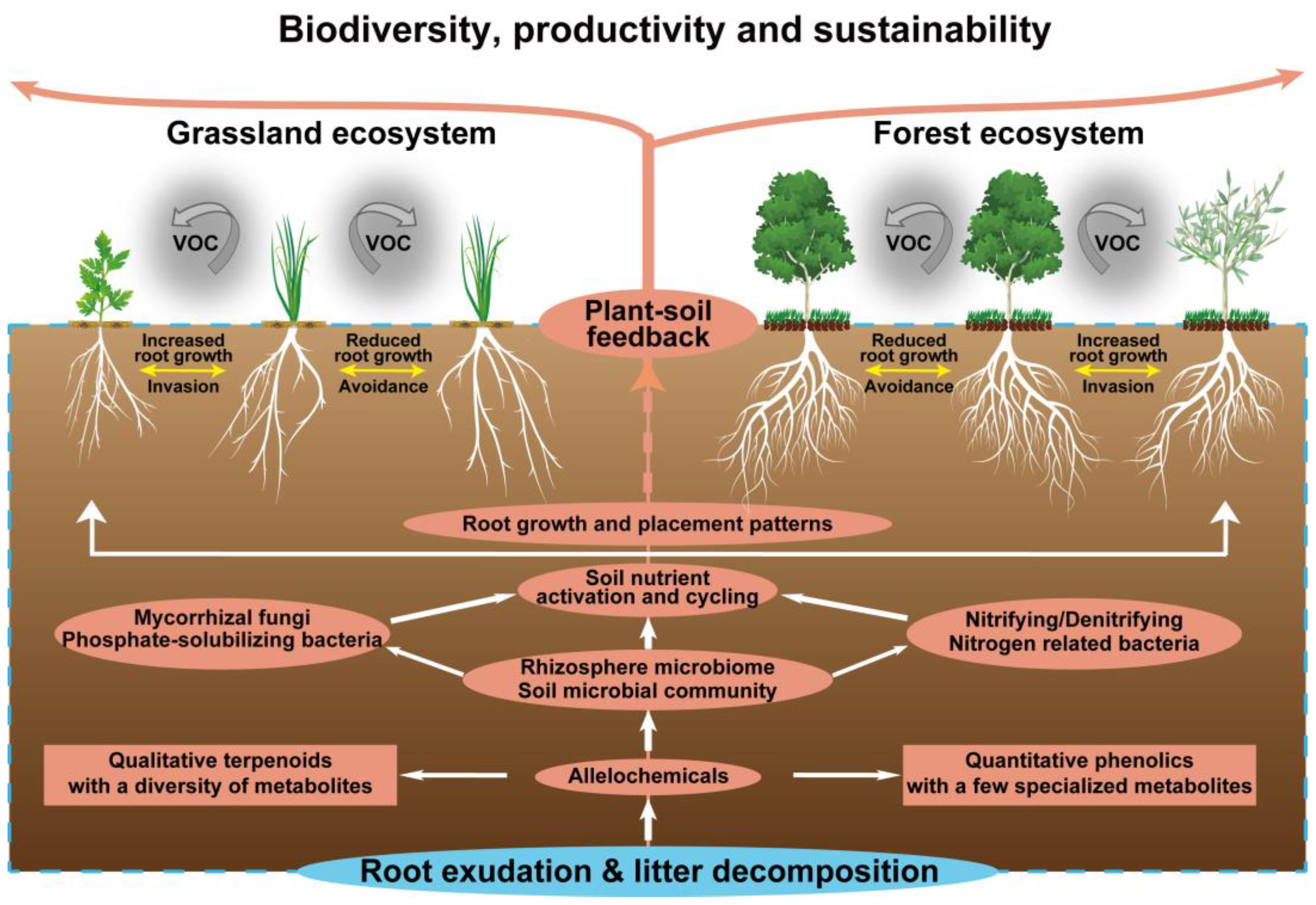This detailed educational illustration, titled "Biodiversity, Productivity, and Sustainability," vividly portrays the intricacies of the grassland ecosystem on the left and the forest ecosystem on the right. The color diagram, utilizing hues of green, white, brown, yellow, beige, and blue, offers a bifocal view of both ecosystems from above ground, displaying plants and trees, and below ground, revealing their extensive root systems. The diagram is distinguished by numerous scientific terms and is meticulously labeled to explain various stages and processes, such as root exudation and litter decomposition, essential for plant growth and soil nourishment. Accompanied by arrows and lines, it details how plant-soil feedback mechanisms operate, illustrating how roots grow and decompose, thereby enriching the soil. The steps and text flowing down the illustration break down complex concepts related to biodiversity, productivity, and sustainability, making it an essential visual for educational purposes.